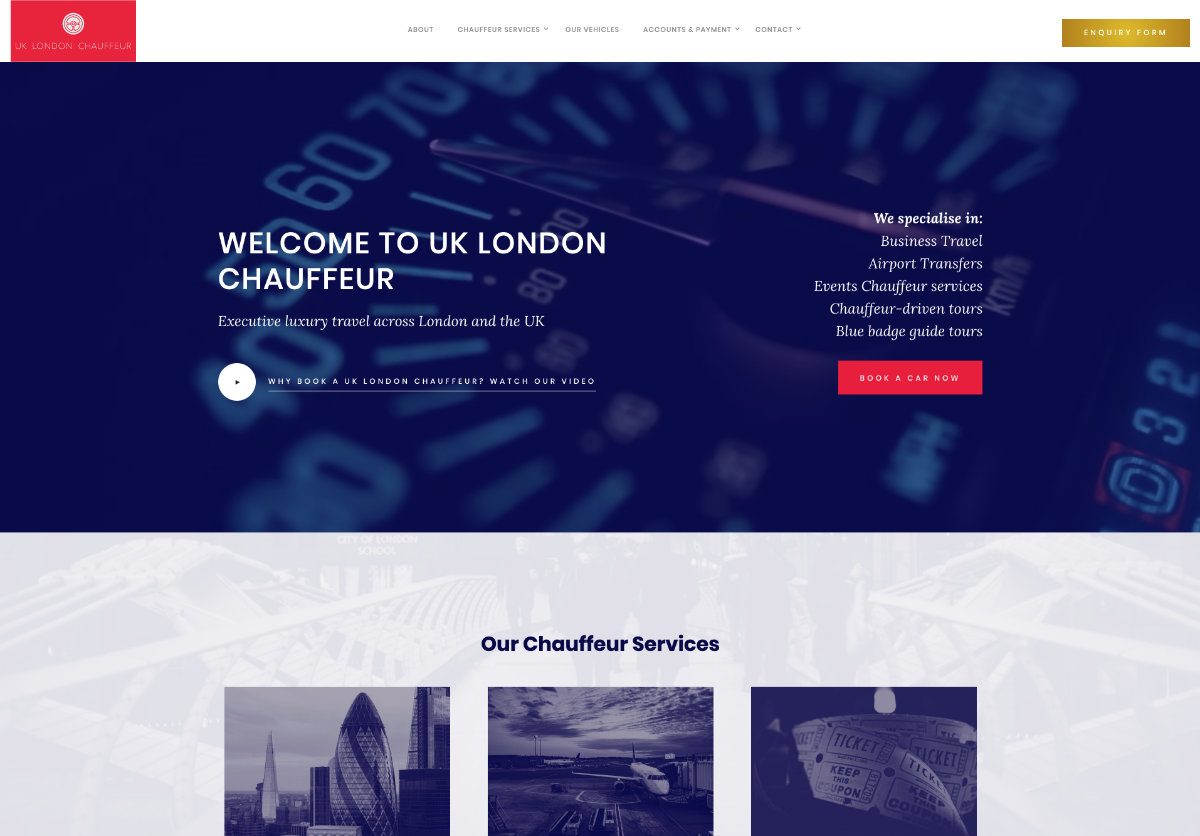This is a detailed caption describing a horizontal rectangular website image:

---

The image is a horizontally oriented rectangular screenshot of a website, primarily showcasing a navy blue and gold design. In the top-left corner, a red tab sticks out, though the text on it is unreadable. Adjacent, to the right of the tab, is a horizontal, rectangular gold graphic, which might contain the words "Inquiry Form," though the text is unclear.

The upper section of the image, taking up more than half of the space, features a navy blue background with all-capital white text that reads: "WELCOME TO UK LONDON CHAUFFEUR." The word "CHAUFFEUR" is directly below the rest of the heading. Beneath this, in a smaller white font, it states: "Executive Luxury Travel Across London and the UK," followed by text that is too small to decipher.

On the right side of this navy blue section, white text lists their specialties: "We specialize in" followed by individual lines that include "Business Travel," "Airport Transfers," "Event Chauffeur Services," "Chauffeur-Driven Tours," and another unreadable term that appears to be related to guided tours. Below this list, there's a prominent red horizontal button labeled "Book a Car Now."

The bottom part of the image features a lighter background with a tone-on-tone design. In this section, it declares "Our Chauffeur Services" in a dark font, paired with three horizontal black and white images depicting various scenes or subjects related to their services.